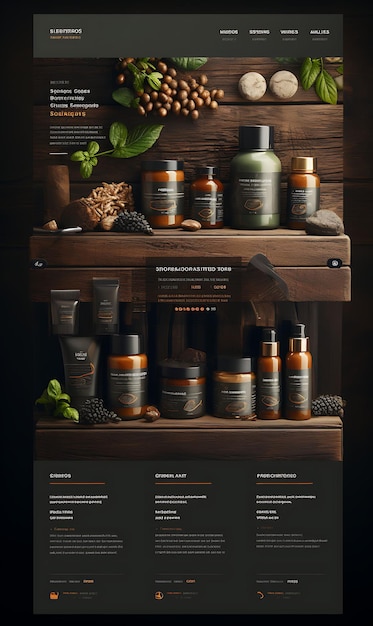The image features an advertisement for healthcare and beauty products displayed on dark chestnut brown wooden shelves. The setup includes two primary shelves, the upper one holding a variety of supplement bottles, among which you can spot containers with red and green contents. The lower shelf is populated with numerous small bottles containing a reddish-brown liquid, identifiable by their black labels. Artistic decorations such as leaves, seeds, berries, and stones are also arranged on the shelves, adding a natural aesthetic.

The image is framed with two thick black stripes on the left and right sides, and thinner black stripes on the top and bottom. An overlay of text in white and yellow can be found on a gray background in the upper corners, consisting of four distinct groupings of text. There are also decorative elements such as green leaves and white circles placed near the top shelf. The products primarily include amber-colored plastic containers with black lids, and one notable bottle with a gold cap. Additionally, there are black squeeze bottles, giving the shelves a cohesive and polished look. The bottom of the page contains more text set against a black background, detailing the product features, although it's too small to read clearly.